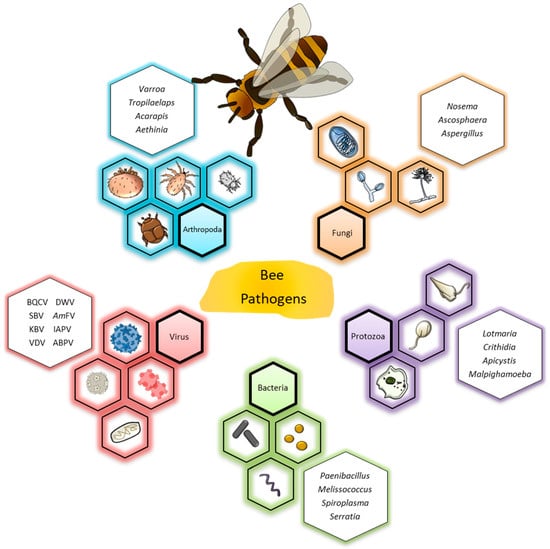This image appears to be a detailed scientific diagram from a biology textbook focused on potential pathogens that affect honeybees. At the top is a drawing of a bee, setting the central theme. In the middle, the heading "Bee Pathogens" stands out against a yellow background with black text. Surrounding this are five color-coded sections, each representing a different category of pathogens.

- In the top right, the blue section is labeled "Arthropoda," listing pathogens such as Varroa, Tropilaelaps, Acarapis, and Athena.
- Adjacent to this, the beige section labeled "Fungi" includes Nosema, Ophiocordyceps, Ascosphaera, and Aspergillus.
- Continuing clockwise, the purple section for "Protozoa" features Lotmaria, Crithidia, Apicystis, and Ophryocystis.
- The green section at the bottom center is labeled "Bacteria," showcasing Paenibacillus, Melissococcus, Spiroplasma, and Serratia.
- Finally, in the bottom left, the red section labeled "Virus" includes several acronyms representing different viral pathogens.

Each section contains both the scientific names and visual depictions of the pathogens, providing a comprehensive overview. The use of color-coding helps to clearly differentiate between the categories, making it a useful educational tool that blends informative content with engaging visuals.